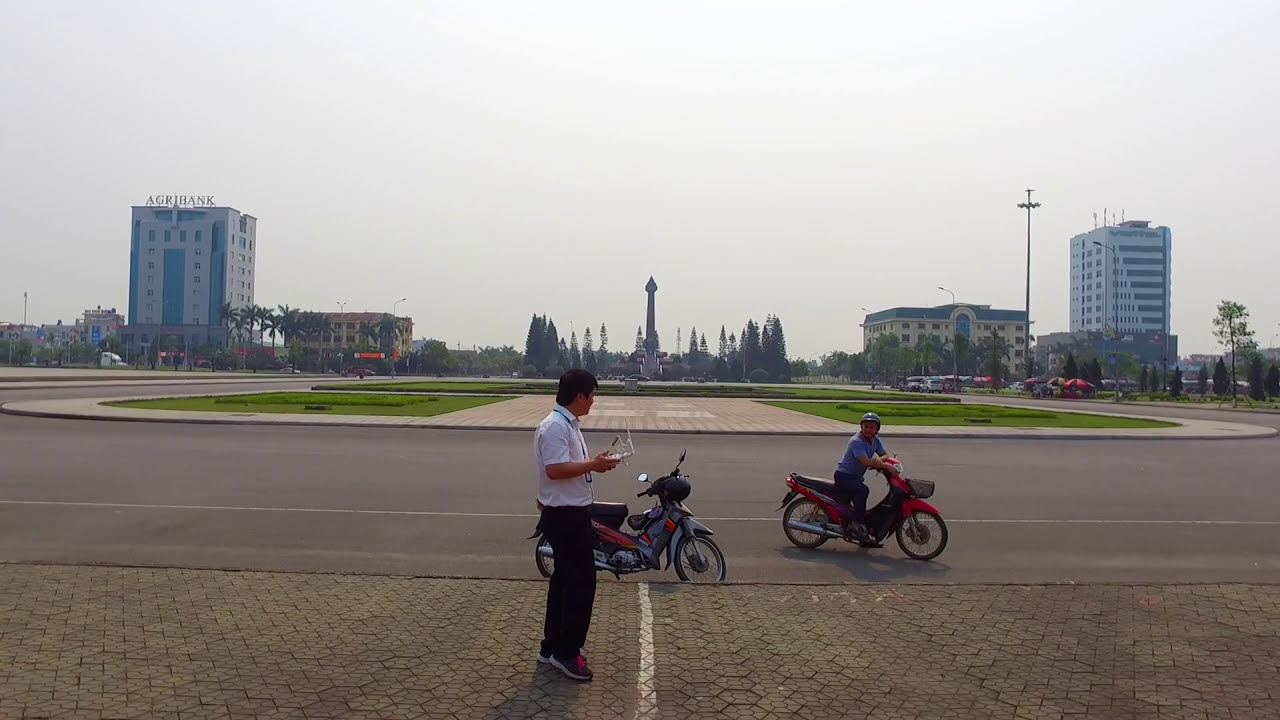The photograph captures an overcast urban scene with two men and their electric motorbikes in the foreground. The sky is gray and hazy, with the sun faintly shining through the clouds above. Dominating the background, tall multi-floor buildings that resemble banks or hotels flank a central tower-like structure resembling a Hershey Kiss, surrounded by trees. Besides these tall edifices, several shorter buildings line either side, creating a layered cityscape.

In the lower foreground, a wide cobblestone sidewalk features prominently. On this sidewalk stands an Asian man with brown skin and short black hair, wearing a white short-sleeved button-up shirt and dark pants. He's holding a piece of paperwork or perhaps a remote control. Facing right, he appears engaged with the second man, who is on a red motorbike parked in the street. This second individual, wearing a helmet, a blue or gray shirt, and dark pants, looks back towards the man on the sidewalk. They could be conversing.

Adding to the scene are various elements like a big pole that appears to be a streetlight, some possible greenery, a fountain with a small tower in the background, and extensive paved surfaces. The image overall portrays a dynamic and bustling urban atmosphere against a muted, smoggy sky.